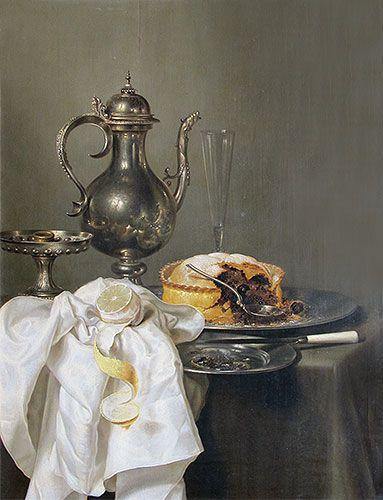This painting is a detailed still life featuring a gray-dominated color palette. In the background, a muted gray sets a somber tone, complemented by a dark gray tablecloth draped over the table. Arranged atop the table are several meticulously depicted items. On the left side, a white cloth partially shrouds a large, partially peeled fruit with a spiral rind revealing its yellowish, citrus interior—its size and dull color suggests it might be an unusually large lemon or perhaps a light-colored orange. 

Central to the composition is an ornate silver teapot, flaunting intricate designs. To its right stands a tall, elegant glass, conical, akin to a champagne flute. Below this arrangement lies a prominent silver platter holding a dessert, possibly a pie or pudding, characterized by a brownish, textured filling. An accompanying silver spoon is positioned next to the dessert, indicating it's been cut into. Directly beneath this platter is a smaller silver plate adorned with a knife, notable for its distinctive white handle.

This scene, reminiscent of a refined tea service setup, captures the essence of an elegantly prepared table ready to serve, blending a classic and inviting atmosphere with meticulous artistry in the portrayal of everyday objects.